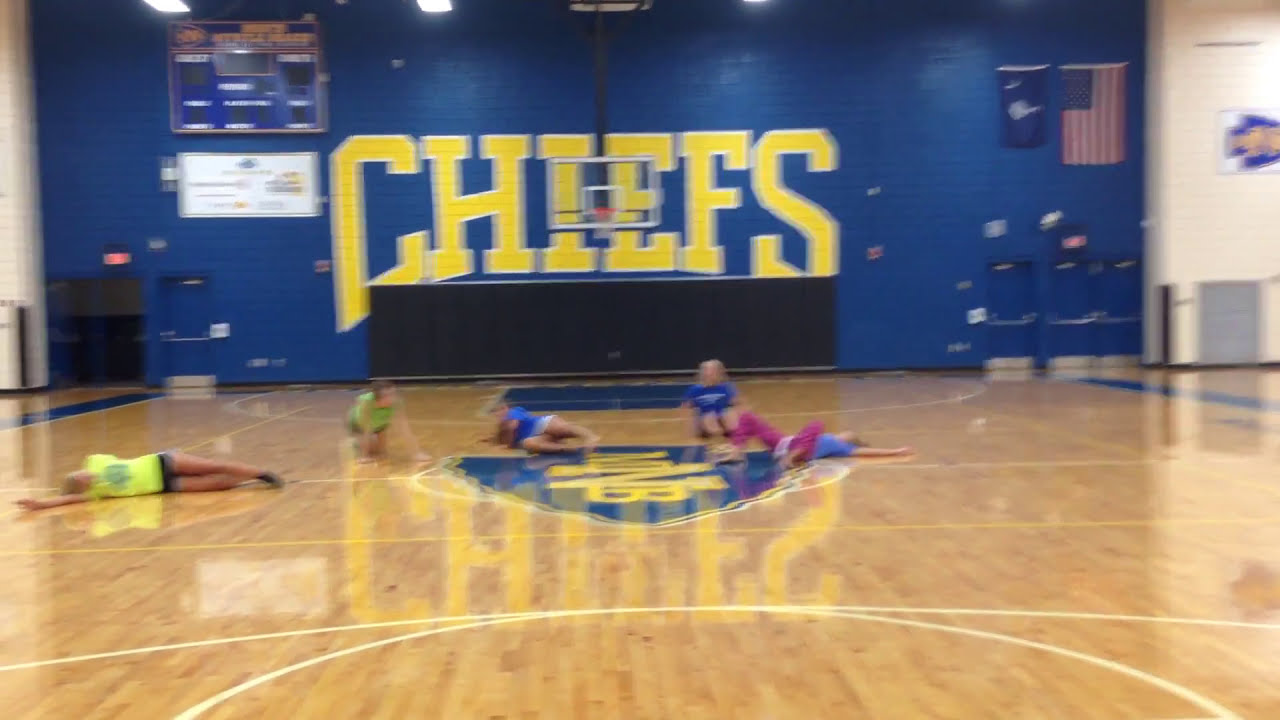The image depicts a slightly blurry high school gymnasium with a shiny hardwood floor marked with traditional lines for basketball and other sports. Prominently displayed on the deep blue back wall is the word "Chiefs" in large, yellow letters with a white outline. Below the "Chiefs" sign is a drop-down basketball hoop. To the left side of the wall, there is a scoreboard, and on the right side, an American flag hangs alongside a blue flag bearing a central image. The gymnasium's glossy floor features a yellow and blue emblem in its center. 

In the image's foreground, five girls of apparent Caucasian descent are scattered on the floor. Two girls on the left are wearing bright yellow shirts with short black shorts; one is lying down with her arm stretched out, and the other is up on all fours. Three other girls to the right are dressed in blue tops; one is lying down with her feet towards the camera, another is sitting facing the camera, and the third, who is wearing pink long pants along with a blue top, is lying diagonally. Additionally, there is a doorway visible on the right side of the gym, with some light sources inset into the ceiling contributing to the floor's glare.